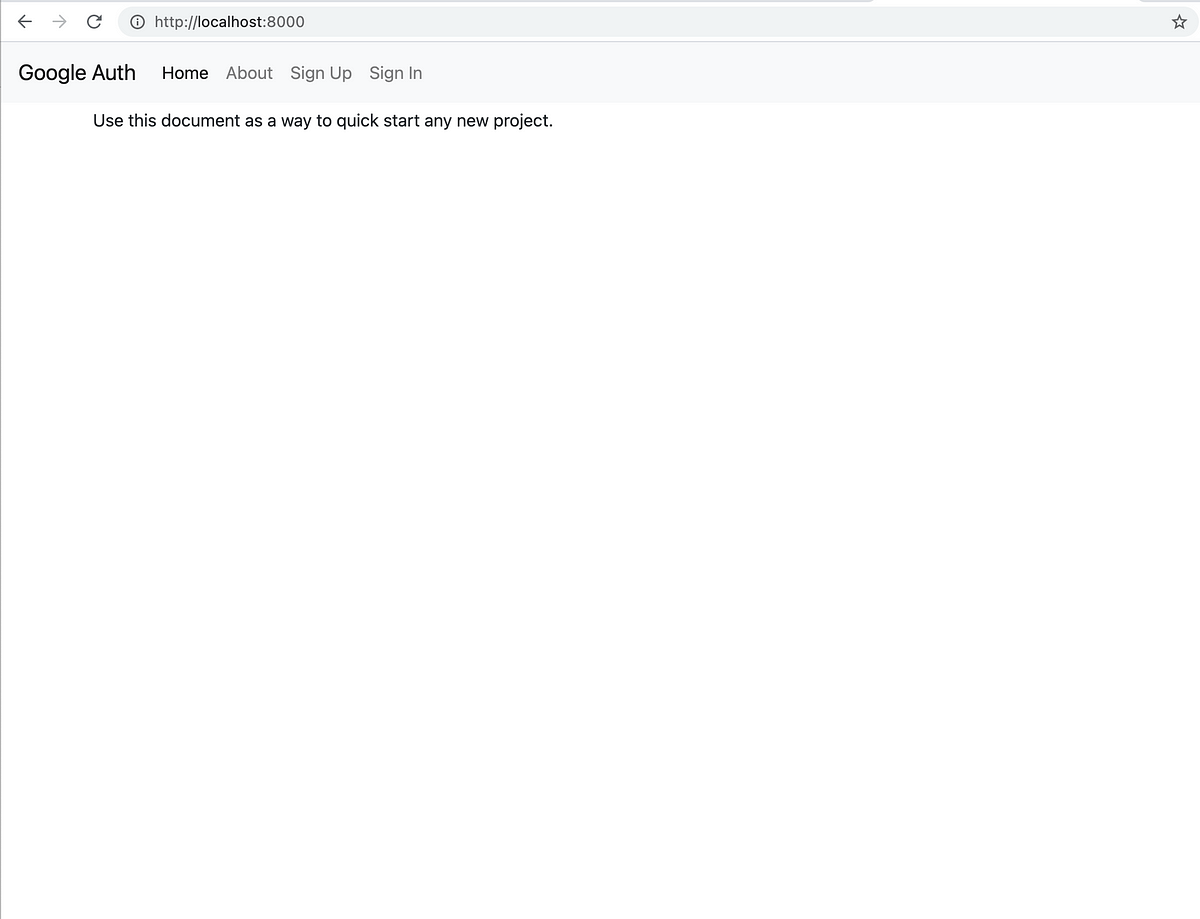This screenshot captures a minimally designed webpage with sparse text and a clean, uncluttered interface. Dominating the top section, the page features a simple navigation bar. In the upper left, there are three small arrows: one pointing left, another pointing right, and a circular arrow, likely for refreshing the page. Adjacent to this, a slightly darker gray background frames an address bar. An informational icon (an 'i' inside a circle) appears at the start of the bar, which reads "http://localhost:8000." Positioned at the far right of the address bar is a star icon.

Directly below the address bar, in large, black text, the words "Google Auth" are displayed, followed by smaller text listing "Home," "About," "Sign Up," and "Sign In." This is the entirety of the navigation menu. Below this, a single line of text states, "Use this document as a way to quick start any new project," indicating the purpose of the page.

Overall, the page is stark and devoid of any other visual elements such as images, additional text, icons, or logos. The absence of content highlights the simplicity and focused functionality of this webpage.